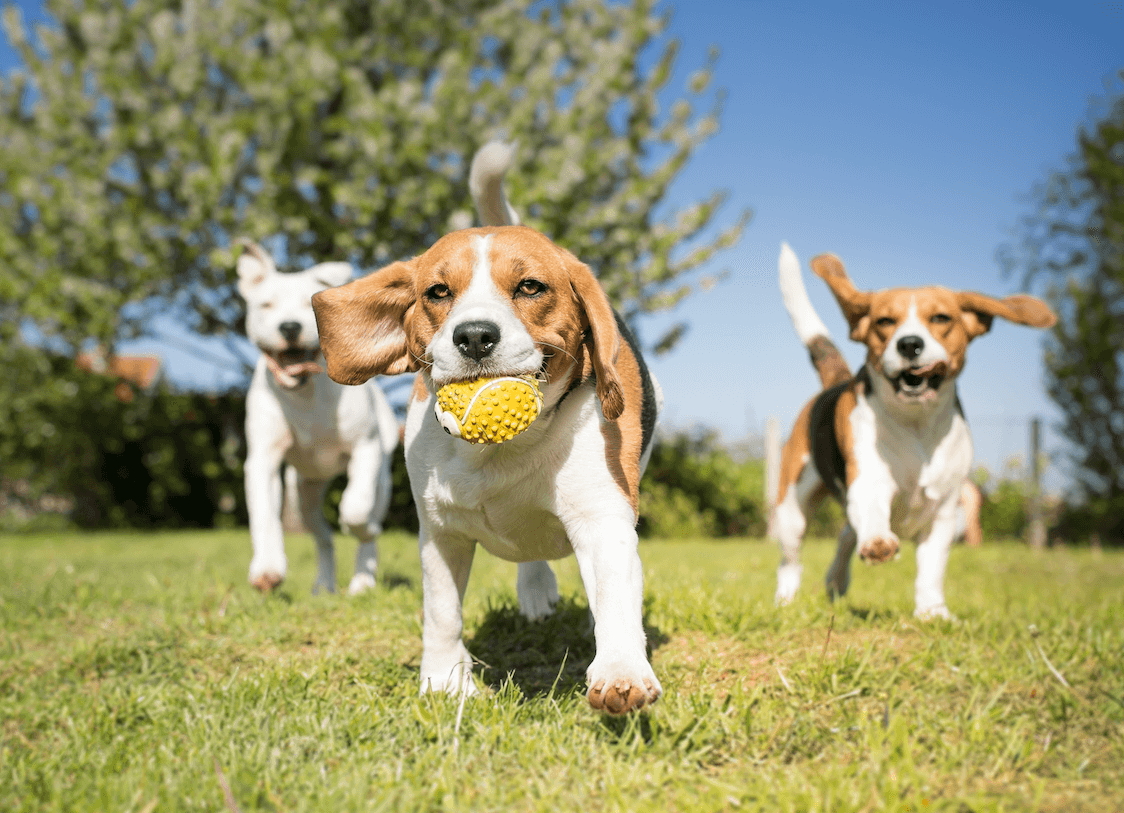In this vibrant photograph taken on a sunny, clear day in a lush green park, three joyous dogs are captured mid-run, racing towards the camera. The lead dog, a brown and white beagle with floppy ears and expressive brown eyes, proudly carries a yellow, googly-eyed puffer fish toy in his mouth. To his right, another beagle, almost identical with its white and brown fur, eagerly bounds forward with its brown ears flopping in the breeze and its white tail held high. On the left, a lively, all-white dog, possibly a pit bull mix, runs with its mouth open and tongue playfully flapping in the wind. The grassy park is adorned with various trees and bushes, and in the background, the sky is a clear, light blue, emphasizing the warm, cheerful atmosphere of the scene.